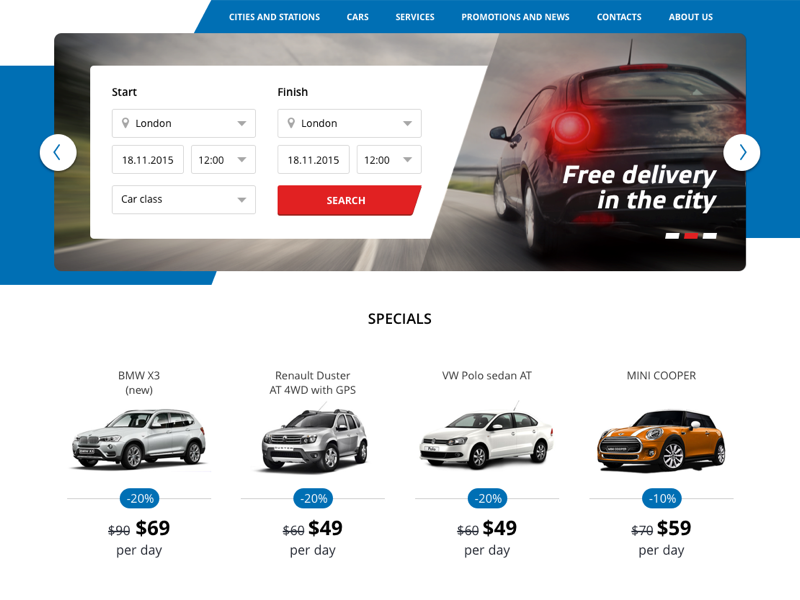This screenshot captures a specific page from an unknown car rental website. At the top, the navigation bar includes options such as "Cities and Stations," "Cars," "Services," "Promotions and News," "Contacts," and "About Us." 

The background image, prominently displayed, features a street view with a black vehicle driving away, its taillights illuminated, adding to the dynamic feel of the page.

On the left side, there's an option section for booking a car:
- Start Location: London
- Start Date: 18-11-2015
- Start Time: 12:00 PM
- Car Class: [Selection]
- Finish Location: London
- Finish Date: 18-11-2015
- Finish Time: 12:00 PM
- A "Search" button is provided along with a note about "Free Delivery in the City."

Below this section, there is a "Specials" section highlighting various promotional offers on car rentals:
1. **BMW X3**: Described as new, with a 20% discount applied. The original price of $90 per day is crossed out, replaced by the new rate of $69 per day. The image shows a silver four-door vehicle.
2. **Renault Duster AT4WD with GPS**: Also offered at 20% off, reducing the daily rate from $60 to $49. This vehicle is a silver four-door SUV.
3. **VW Polo Sedan AT**: Available at a 20% discount, bringing the price down from $60 to $49 per day. The image depicts a white four-door car.
4. **Mini Cooper**: Offered at a 10% discount, lowering the price from $70 to $59 per day. The image shows an orange two-door vehicle.